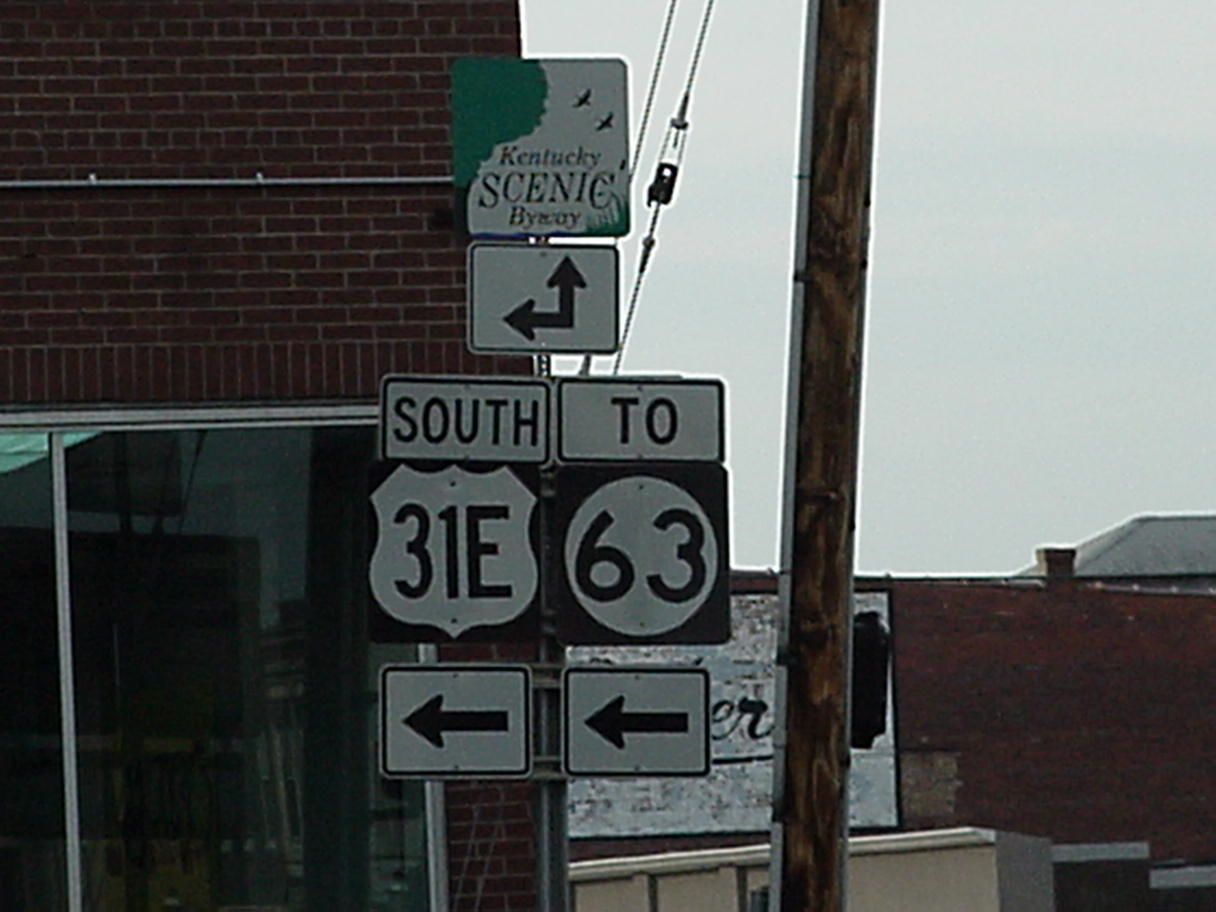In the outdoor scene, the top right corner showcases a gray, overcast sky. In the top left, there is a brick wall, with the bricks separated by layers of cement. A prominent silver pole cuts through the image vertically. Toward the bottom left, a smaller pole with a metallic feature at the top stands out, intersecting with wires that stretch across the skyline. 

A variety of signs populate the scene: a white sign with a black arrow pointing upwards, another black arrow pointing left, and a sign denoting "Kentucky Scenic" among other text. The bottom of the image features a sign with an arrow pointing left. Green and red birds can be seen perched to the right. Additionally, a sign in the top left directs possibly to "South," while numbers "2," "31 to 8," and "63" are displayed on respective signs throughout the scene.